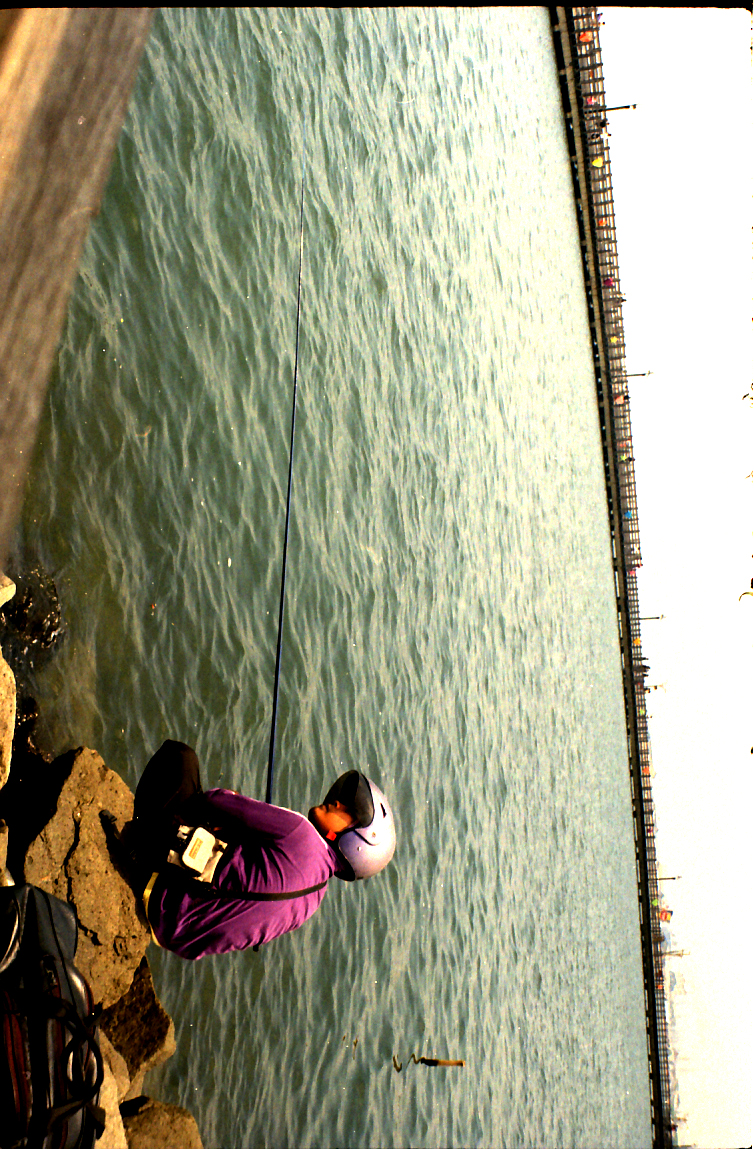In this sideways-oriented photograph, a person with darker skin, possibly of Hispanic or Asian descent, is seen crouching on a rock near a large body of water, possibly the ocean. They are wearing a purple long-sleeved shirt, black pants, and a silver helmet with a black visor. The person appears to be fishing, holding a fishing pole out over the water. The bright, white sky suggests a sunny yet cloudy day. In the background, a pier spans from the top to the bottom of the image due to its tilted perspective. The pier is populated with colorful objects—perhaps signs—in hues of orange, red, yellow, blue, and green, and may have some poles along its length. There might also be people walking on this pier, adding to the activity of the scene. Some shore is visible in the upper left corner of the photograph, further grounding the setting.